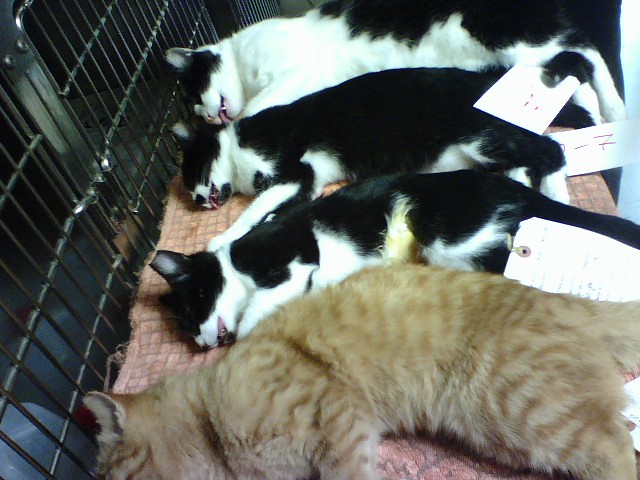The image depicts a deeply unsettling and tragic scene of four deceased cats lying inside a black metal cage with a reddish-brown blanket underneath them. Each cat has a tag attached to its tail, indicating they have been cataloged. The cats are positioned horizontally and appear lifeless, with their mouths open and tongues hanging out, adding to the heart-wrenching imagery. 

At the bottom of the photo is a light beige cat with darker brown stripes, partially curled. Above it, three black and white cats are resting side by side. The cat at the very top of the image noticeably has its tongue protruding from its open mouth. Their lifeless bodies and the stark black cage create a profoundly disturbing and sorrowful visual.